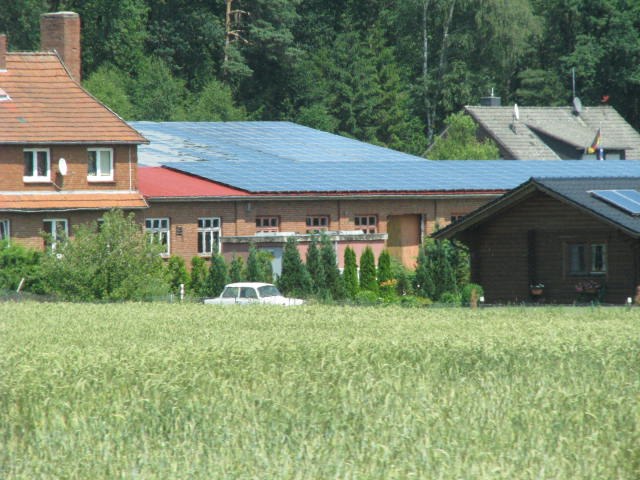A photograph captures a rural neighborhood scene, featuring a mix of buildings and natural elements. In the foreground, there is a vibrant field of tall, green grass that stretches towards a collection of attached homes and additional structures. 

Dominating the scene is a sprawling, single-story building composed of red brick, adorned with a flat metal roof partly obscured by solar panels. To the left, a portion of this structure rises to two stories, showcasing an A-frame roof equipped with antennas. Adjacent to this building on the right-hand side, another single-story house stands out with its dark brown wooden exterior and black, A-frame roof also fitted with solar panels.

Parked in front of these buildings on the far side of the field is a small, white automobile, likely an older four-door sedan from the 1970s. The scene is framed by a dense forest of tall, dark green trees and bushes that stretches up a hill, creating a natural backdrop for the homes. In the distance, additional homes can be seen peeking through the thick foliage, completing the rustic and serene landscape.